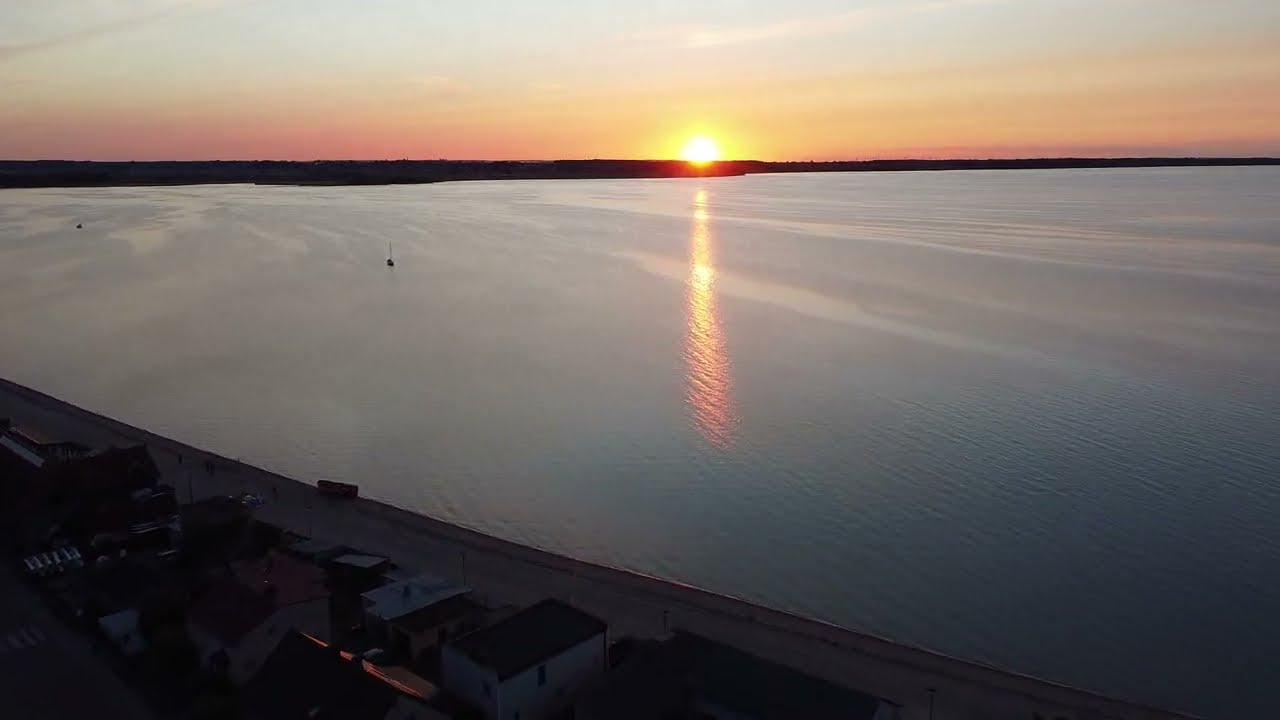This photograph captures a stunning sunset over a vast expanse of calm, blue-gray ocean. Taken from an elevated vantage point, possibly from a hotel balcony, the image reveals a serene landscape where the sky meets the water, forming a vivid horizon. The setting sun, almost blindingly white at its core, is surrounded by a breathtaking palette of pink, orange, yellow, and purple hues, which seamlessly blend into each other and reflect off the tranquil surface of the ocean. In the image's lower left corner, small beach houses can be discerned, with one house in particular standing out with its white walls and black roof. A road runs diagonally in front of these houses. The presence of distant hills silhouetted against the glowing sky adds further depth and tranquility to this mesmerizing scene.